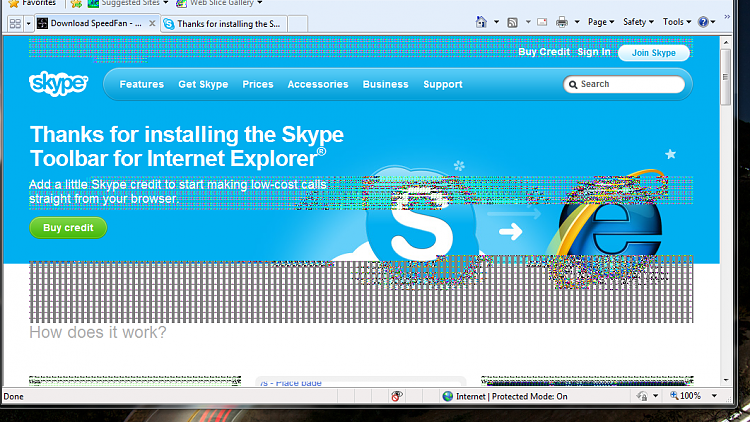The image is a screenshot of a website, likely depicting a web browser interface. The screenshot is approximately 50% wider than it is tall. At the top of the image, there is a menu bar. In the upper left corner, there's a yellow star icon labeled "Favorites," followed by menu options: "Suggested Sites" and "Web Slice Gallery," suggesting these are sections within a Favorites menu.

Moving further down, the browser appears to have two open tabs. The first tab is labeled "Download Speed Fan," and the second tab features the Skype logo with the text "Thanks for Installing S," likely referring to Skype.

The main content of the screenshot focuses on the Skype webpage. The top two-thirds of the page feature a light blue background with the Skype logo positioned in the upper left corner. To the right of the logo, there are several white text menu options: "Features," "Get Skype," "Prices," "Accessories," "Business," and "Support." On the far-right side, there's a search bar.

Beneath the header, in prominent white text, the page displays the message "Thanks for Installing the Skype Toolbar for Internet Explorer." Below this message, in smaller text, it encourages users to "Add a little Skype credit to start making low-cost calls straight from your browser." A green button below this smaller text is labeled "Buy Credit" in white text. On the right side of the banner, there is a sequence of icons: the Skype logo, a right arrow, and the Internet Explorer icon.